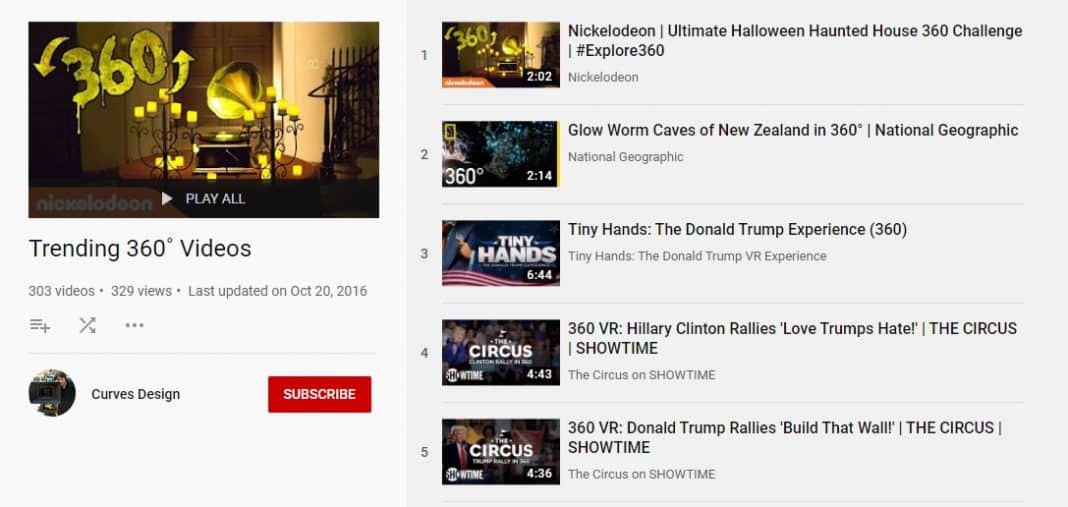**Trending 360-Degree Videos Overview:**

1. **General Information:**
   - **Total Videos:** 303
   - **Total Views:** 329
   - **Last Updated:** October 20th, 2016

2. **Video Descriptions:**

   - **Curves Design:**
     - **Content:** A man playing the piano.
     - **Visual Cue:** A red "Subscribe" button.
     - **Background:** Gray.

   - **Nickelodeon Ultimate Halloween Haunted House 360 Challenge:**
     - **Hashtag:** #Explore360
     - **Visual Description:** A room adorned with gold balloons.
     - **Associated Brand:** Nickelodeon.

   - **Glow Worm Caves of New Zealand by National Geographic:**
     - **Duration:** 2 minutes and 14 seconds.
     - **Content:** Exploration of glow worm caves with luminescent creatures inside.

   - **Tiny Hands, the Donald Trump VR Experience:**
     - **Duration:** 6 minutes and 44 seconds.
     - **Content:** Virtual reality experience related to Donald Trump, labeled as "Tiny Hands."

   - **Hillary Clinton Rallies - "Love Trump's Hate" from The Circus on Showtime:**
     - **Duration:** 4 minutes and 43 seconds.
     - **Content:** Coverage of Hillary Clinton’s rallies showcasing the "Love Trump's Hate" theme.

   - **Donald Trump Rallies - "Build That Wall" from The Circus on Showtime:**
     - **Duration:** 4 minutes and 36 seconds.
     - **Content:** Footage of Donald Trump’s rallies emphasizing the "Build That Wall" slogan.

**Note:** This overview captures the essence and details of the trending 360-degree videos as of the last update in October 2016.